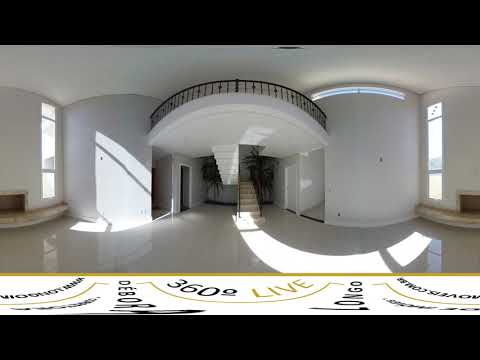This detailed 360-degree panoramic photograph showcases a pristine, unfurnished white living room bathed in sunlight. The image, taken by a 360 camera and labeled "360-degree live" at the bottom, features curved walls due to its panoramic nature. The living room has white ceilings, walls, and a gray floor, all contributing to a clean, minimalist aesthetic. Floor-to-ceiling windows allow ample sunlight to flood the space, casting intricate shadows on the reflective stone or marble floor. On either side of the room, brown wainscoting adds a touch of warmth and contrast. In the center, a balcony with a black wrought-iron railing commands attention, accessible via a staircase that ascends and turns back on itself. A fireplace can be seen on the left side, hinting at the room’s potential for coziness. The overall setting evokes a high-definition, Miami-esque atmosphere, perfect for commercial showcases.